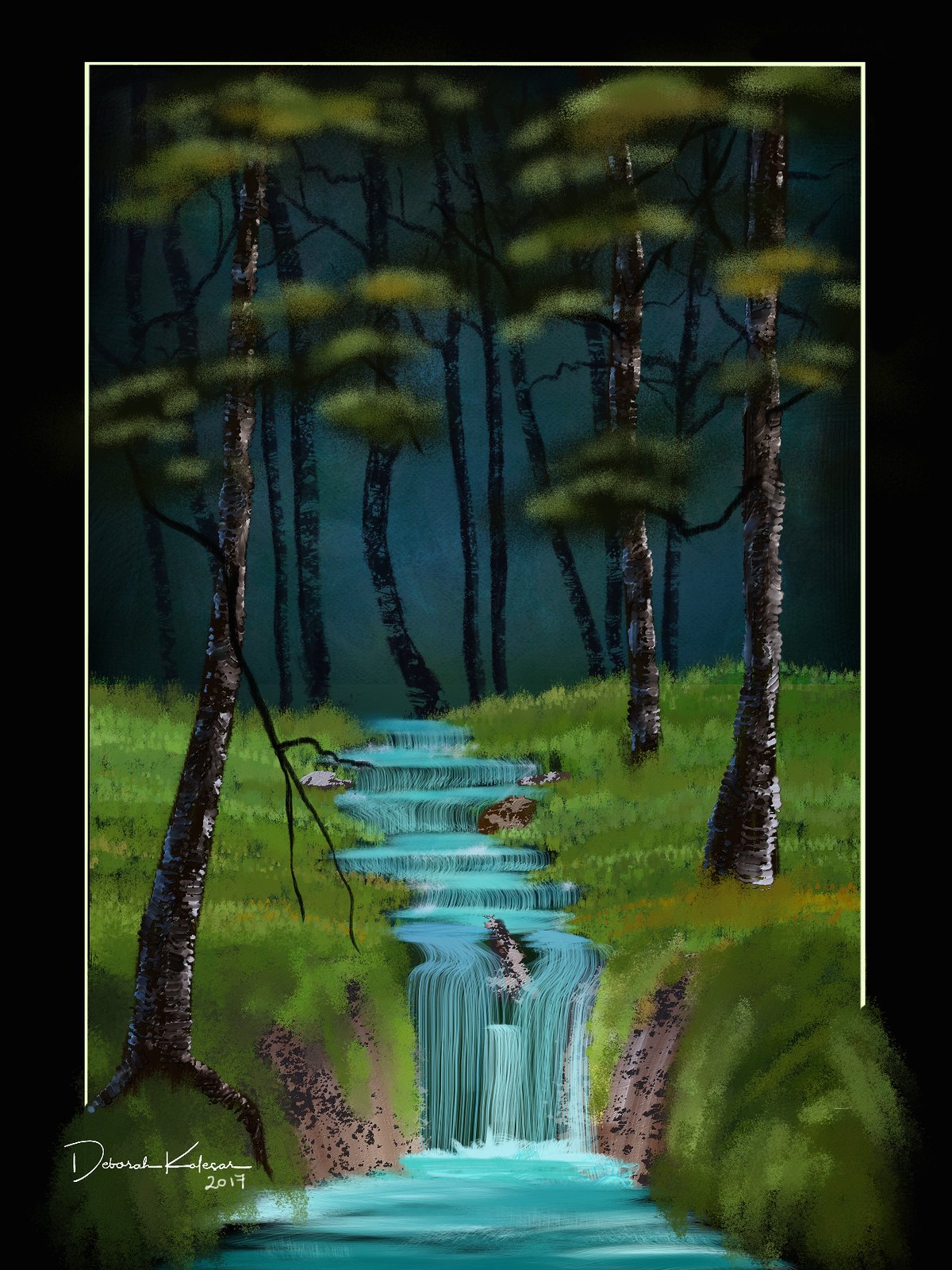The image depicts a detailed and perhaps digitally created painting of a serene natural scene. A winding, small blue creek flows from a distant hill in the background towards the foreground, where it features multiple small waterfalls and one larger waterfall, before opening into a calm retaining pond. The creek is highlighted with white lines indicating movement, especially at the waterfalls where the water crashes. Flanking the creek, the field is covered in tall, alternating patches of light and dark green grass. Sparse trees with dark, camouflage-patterned bark in shades of black and gray stand on either side of the stream, their branches adorned with diffuse, bushy leaves. The painting has a dark, almost deep purple backdrop and is bordered by a thin white line inside a thicker black edge. There is a small, yellowish diffuse patch in front of a tree on the right side of the image. Additionally, there's an artist's signature in the bottom left corner: the first name starts with a 'D' and the last name with a 'K,' dated 2017.